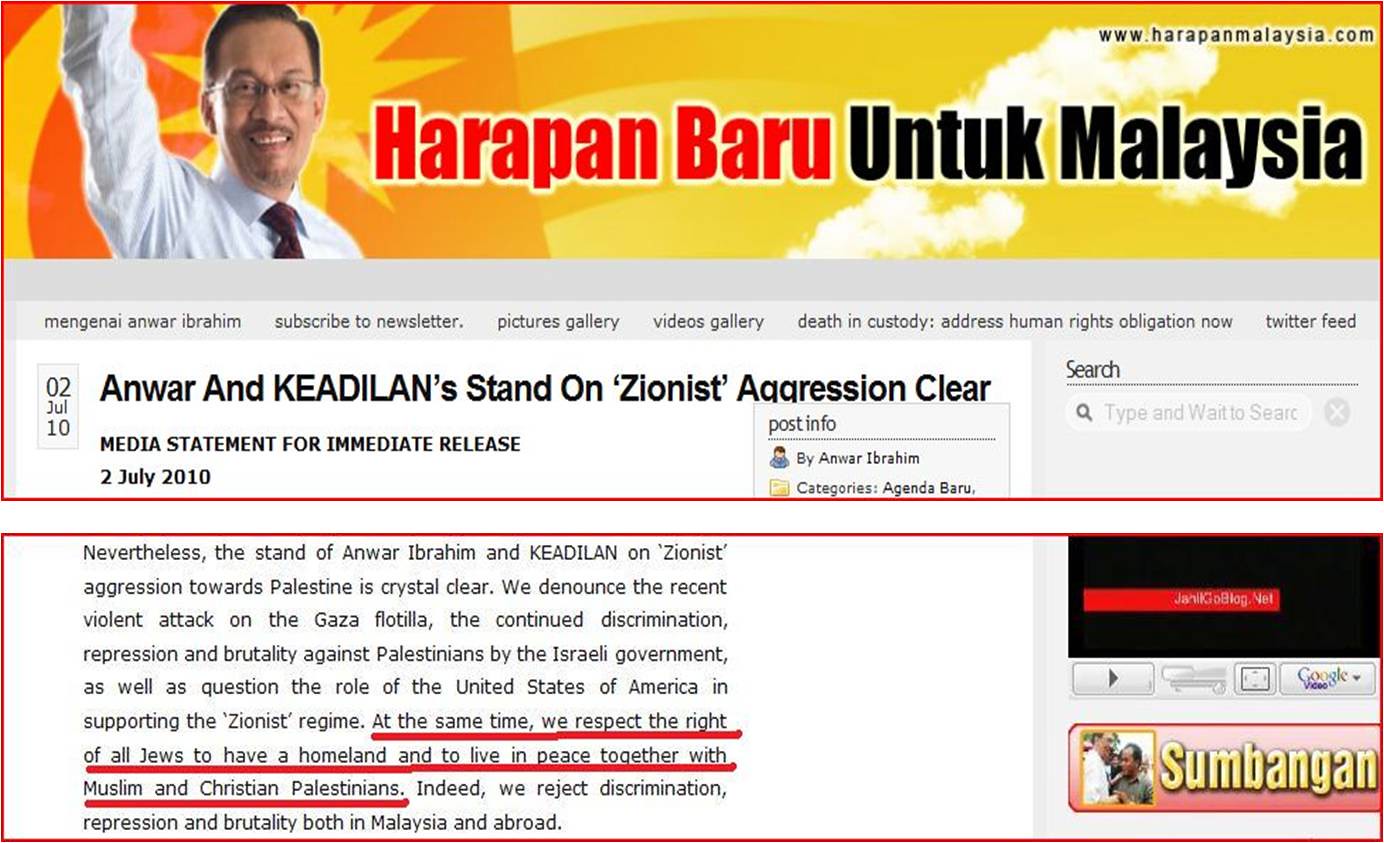The image shows a screenshot of an old website with a banner at the top that reads "Harapan Baru Untucked Malaysia," with the URL www.harapanmalaysia.com displayed just above it. The banner also features an image of an Asian man in a white button-down shirt, a black tie, and glasses. 

The main section of the screenshot contains a post dated July 2nd, 2010, titled "Anwar and KeADILan Stand on Zionist Aggression Clear." The headline appears to be addressing a media statement from Anwar Ibrahim and KeADILan, denouncing Zionist aggression towards Palestine. The text mentions the condemnation of the violent attack on the Gaza flotilla and ongoing repression and brutality against Palestinians by the Israeli government, while also questioning the role of the United States in supporting the Zionist regime. Highlighted, with a red underline, is a statement affirming the right of all Jews to have a homeland and to live in peace with Muslim and Christian Palestinians. 

To the right of the article is a small, old Google video player with a link to something called "Sumbangan" which features an embedded image. Additionally, the website has several navigational links including options like subscribing to a newsletter, accessing a picture gallery, and viewing a Twitter feed. 

The website appears outdated not only in design but also in its use of older multimedia elements and link structures.